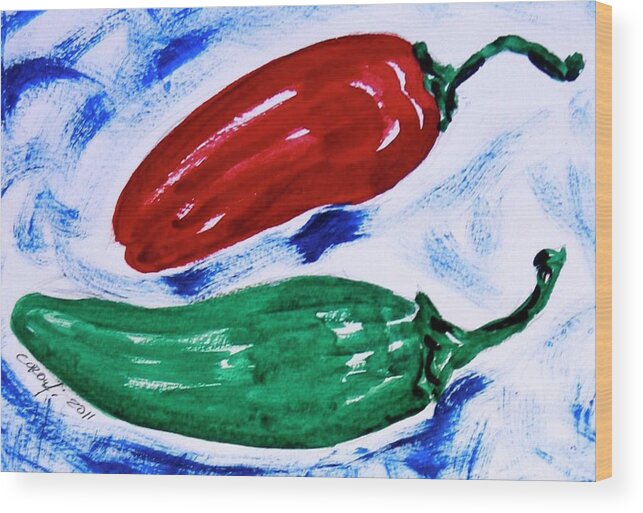This rectangular painting, approximately 5 inches wide and 4 inches high, features two vividly rendered chili peppers against a textured background. The painting is done on what seems to be a wood block, with a light brown wooden edge visible on the right side, giving it a three-dimensional look. The background is an artful blend of off-white and swirling strokes of dark and light blue, applied with a free and expressive brush technique.

At the top of the painting, there is an elongated, glossy red pepper positioned horizontally and slightly angled toward the middle left. It has subtle horizontal indentations and a prominent dark green stem attached to its top right. Below it lies a mixed green pepper, also elongated but wider on its right side and narrowing towards the left with a smooth rounded end. This pepper's green hue contains touches of white, adding texture and depth, and it also sports a dark green stem at the right. 

Both peppers have curved and slightly twisted stems, enhancing the naturalistic feel of the artwork. On the lower left side, just below the green pepper, the artist signed the piece as "C.C. Ralph 2011." This detail adds a personal touch to the vibrant, color-painted wall art, capturing its creation year. The painting’s overall style combines realistic pepper depictions with an abstract, expressive background, making it a striking and immersive visual experience.